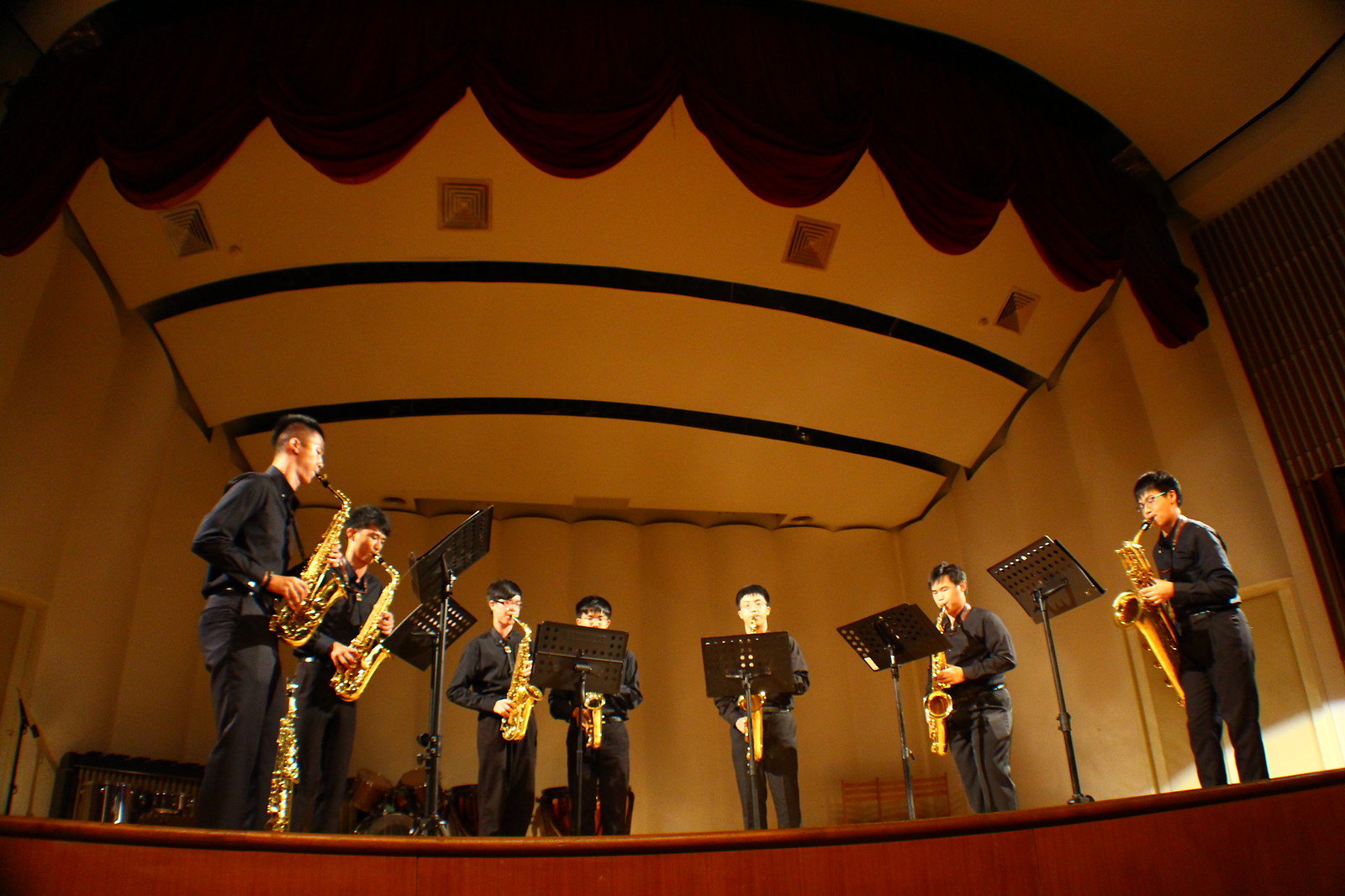The image depicts a mid-20th-century indoor concert hall with a white stage set against a yellowish-brown background. On this stage, seven Asian individuals are performing, each playing different types of saxophones such as baritone, bass, tenor, and alto. These musicians are standing in a semi-circle formation, indicative of an active performance. They are all dressed in black and are using high-quality black music stands, with sheets of paper visible on them. 

The stage is small and acoustically optimized, featuring a decorative dark curtain at the top and a red curtain that is partially drawn up. The ceiling has distinctive black stripes across air conditioning vents reminiscent of the 1950s or 60s, and there are golden squares with crisscross patterns. Additional musical instruments, like drums, can be seen pushed against the wall in the background. The overall scene suggests a dynamic and intimate concert setting.